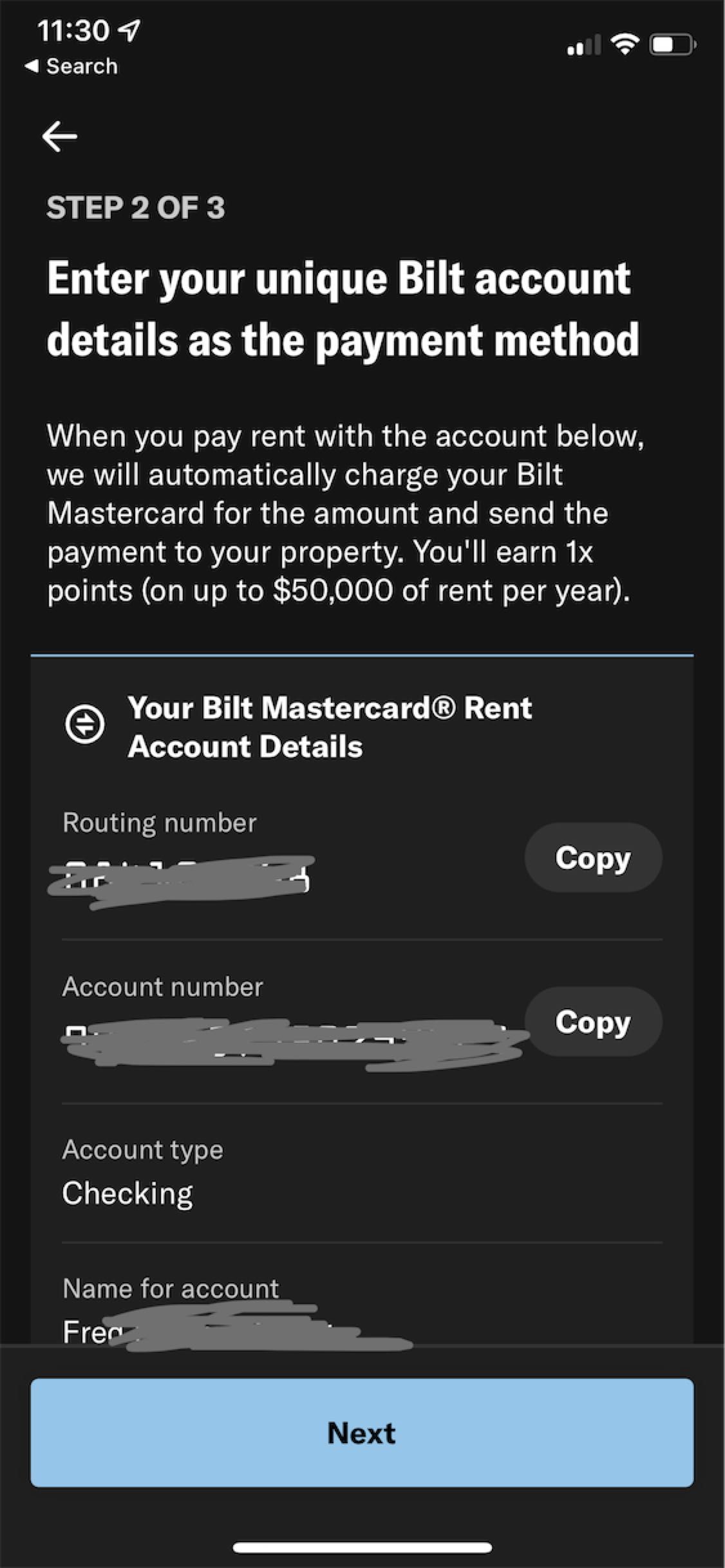The image depicts a smartphone screenshot with a black background. The top of the screen displays the time as 11:30, accompanied by a Telegram icon, a signal strength indicator showing 2 out of 4 bars, a Wi-Fi icon, and a battery icon indicating a half charge. Just below these icons, an arrow points to the left with text reading, "Step 2 of 3". The detailed instructions below advise users to enter their unique Built account details for the payment method. It explains that when users pay their rent using the specified account, their Built MasterCard will be automatically charged for the amount, and the payment will be sent to their property. Users are informed they will earn 1x points on up to $50,000 of rent per year.

Below this, the screenshot outlines fields for "Your Built MasterCard and your rent account details," though all sensitive information such as the routing number, account number, and name for the account has been obscured in gray. Each concealed field features a corresponding "Copy" button. The account type is listed as "Checking," and at the very bottom of the screenshot is a blue button, whose function is not specified.